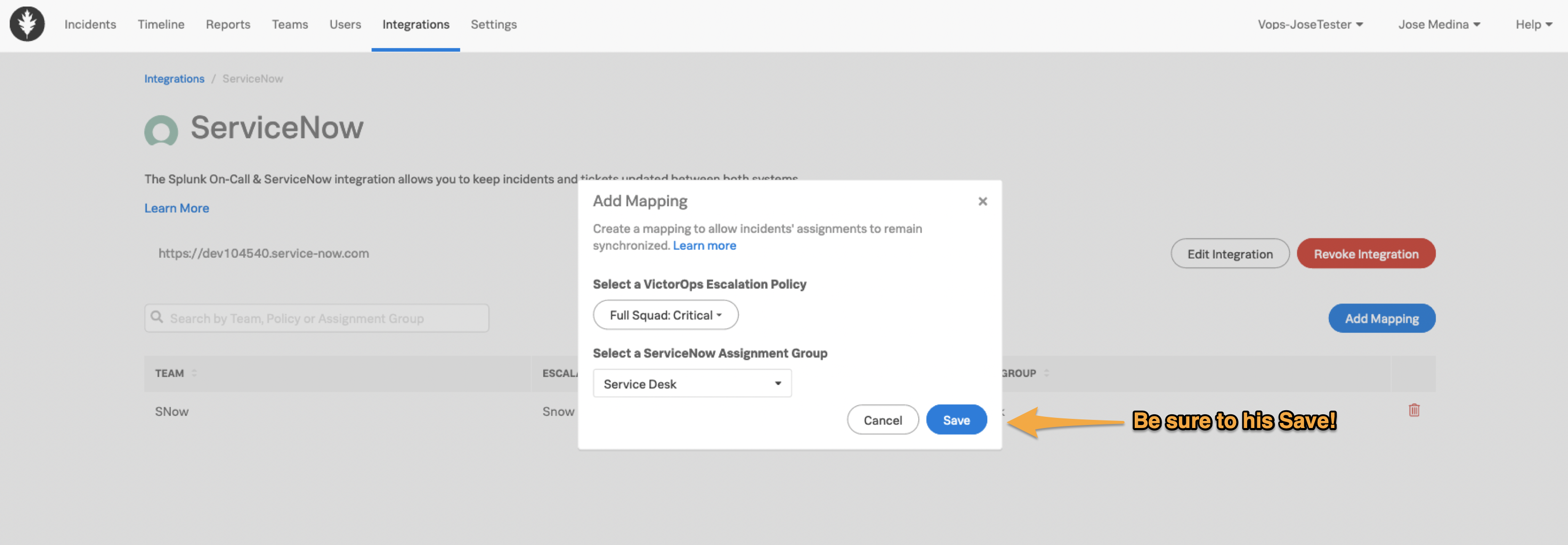This image depicts a web page interface for a technological platform focused on incident and ticket management integration. In the upper right corner, the header reads, "V-O-P-S Jose Tester, Jose Medina, Health." On the top left, there is a black circle containing a leaf icon, followed by a horizontal menu with the options: Incidents, Timeline, Reports, Teams, Users, Integrations (which is underlined), and Settings.

Directly below this menu, the header "Integrations: ServiceNow" is displayed. The accompanying text explains that the integration between Splunk OnCall (formerly VictorOps) and ServiceNow allows for synchronized updates of incidents and tickets across both systems. Additional instructional text reads, "Learn more."

In the center of the page, a white rectangle contains a prompt that states, "Add Mapping. Create a mapping to allow incident assignments to remain synchronized. Learn more." Below this prompt are two dropdown menus. The first asks to "Select a VictorOps Escalation Policy," with "Full Squad Critical" selected. The second prompts the user to "Select a ServiceNow Assignment Group," with "Service Desk" chosen.

At the bottom of this section are two buttons: "Cancel" and "Save." A yellowish-orange arrow points to the "Save" button with nearby text in the same hue that incorrectly reads "His Save" instead of "Hit Save." Beside these options, there are additional buttons for "Edit Integration," a red "Revoke Integration," and a blue "Avoid Mapping."

Finally, at the bottom right of the page, there is an icon of a red trash can.